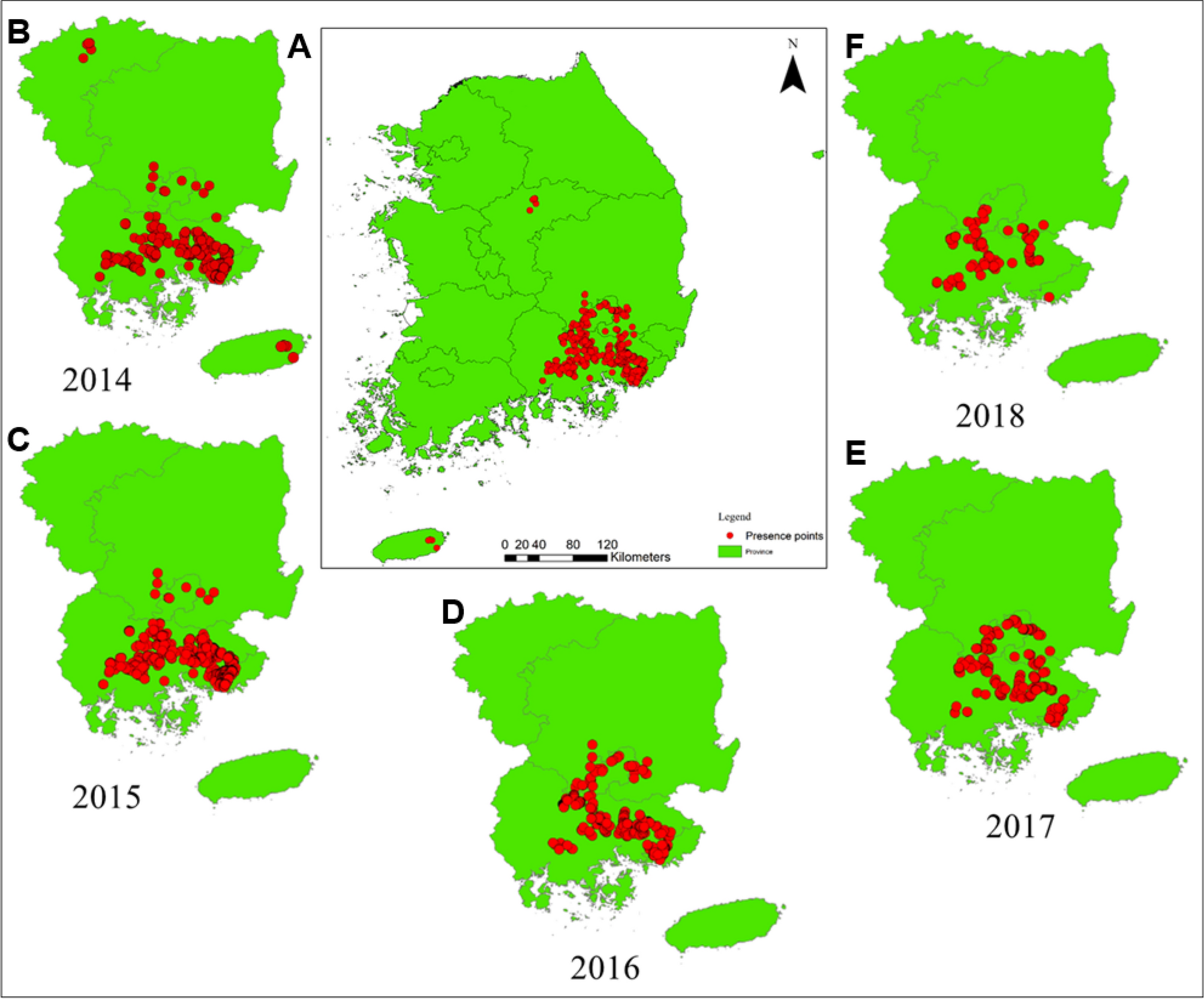The diagram consists of six bright, fluorescent green maps labeled A through F, each enclosed in black squares and featuring clusters of red dots. Map A is centrally positioned and shows red dots densely clustered, especially at the top. Below it, map D is labeled 2016. To the upper left of A, map B is labeled 2014, showing red clusters predominantly toward the top. In the lower left, map C is dated 2015 and exhibits a significant concentration of red dots. Map E, situated in the lower right corner and dated 2017, depicts a small grouping of red dots. Map F, in the upper right, labeled 2018, shows the red dots nearly disappearing. Each map section, while appearing similar to regions like South Korea, likely represents different portions of the same study area or closely related regions, providing a clear and brightly lit view spanning from 2014 to 2018.